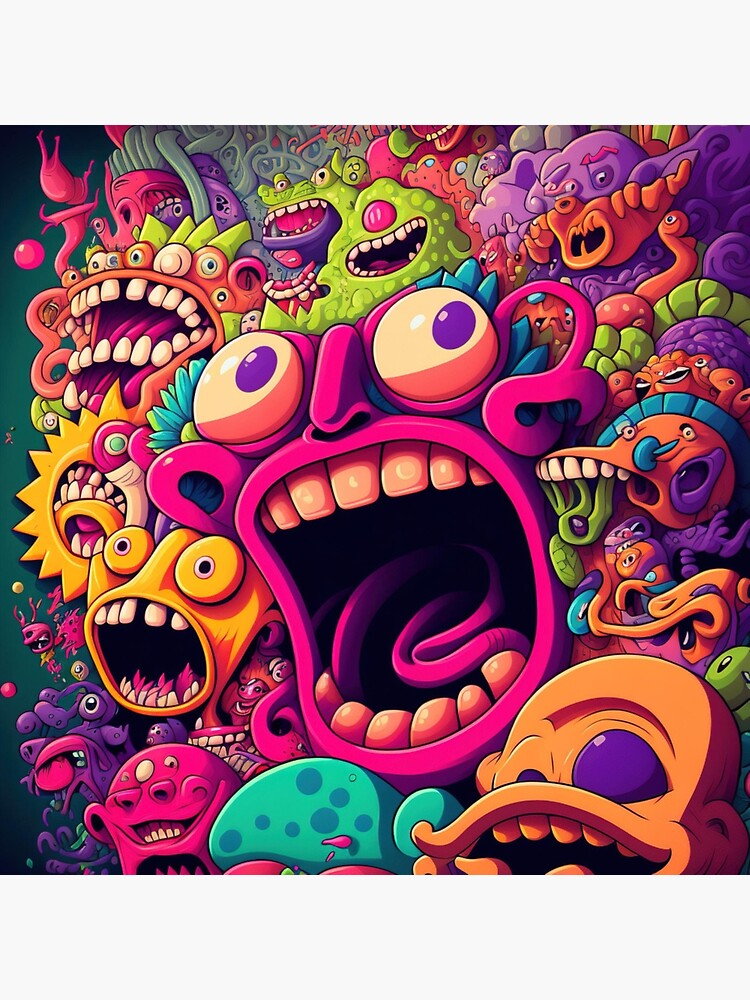This is a vibrant digital illustration rendered in full color, depicting a series of surrealist faces with their mouths agape. At the center of the composition stands the largest face, painted in a striking pink hue. It is adorned with an array of blue hair or possibly flowers, and its wide-open mouth reveals detailed teeth and a tongue. The face also features intriguing purple eyes that add to its otherworldly appearance.

Surrounding the central figure are smaller faces, each unique and vividly colored in shades of yellow, teal, pink, purple, orange, and green. These faces resemble fantastical monsters; some have multiple eyes, while others are cyclopean or possess alien-like characteristics. All of them appear to be gazing directly toward the viewer, enhancing the surreal and slightly unsettling vibe of the piece.

The backdrop of this mesmerizing scene is a dark, tealy green color visible on the left side of the artwork, adding a contrasting depth that complements the vivid hues and bizarre shapes of the faces.